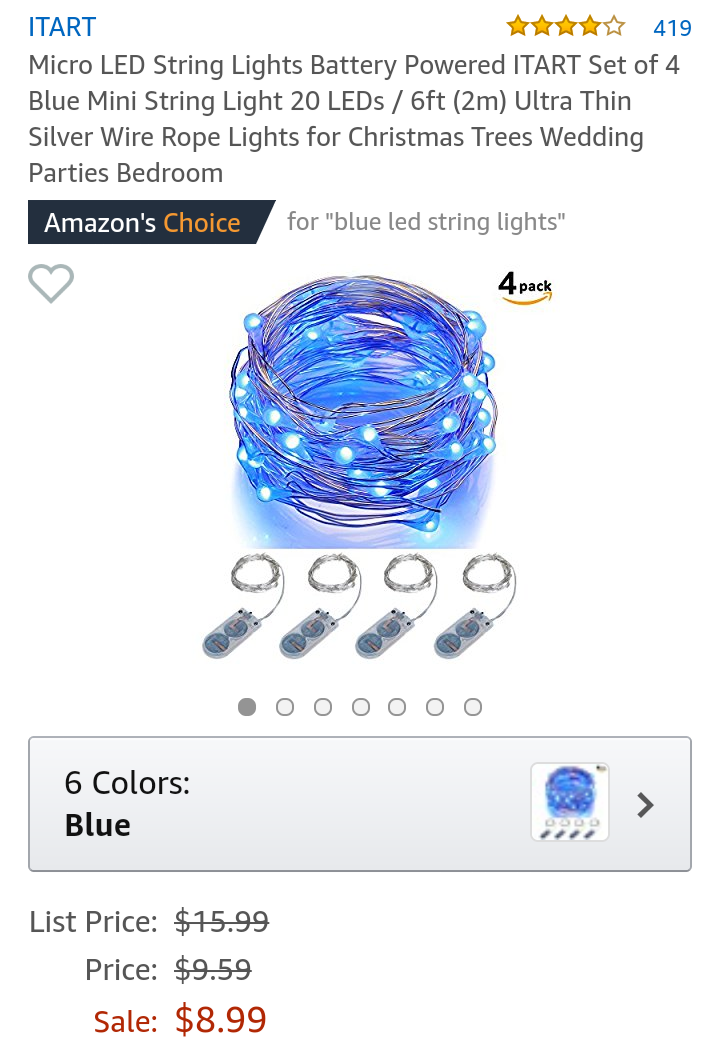A vertical image appears to be a screenshot from an Amazon product listing. At the top, the listing title prominently features the brand name "ITART" in blue capital letters. On the right side, a star rating system shows four out of five stars filled in yellow, with the number "419" in blue indicating the number of reviews.

The main product description reads in black text: "Micro-LED string lights, battery-powered, ITART set of 4 blue mini string lights, 20 LEDs / 6FT (2M), ultra-thin silver wire rope lights for Christmas trees, wedding parties, bedroom." Beneath this, there's a black trapezoidal box with slanted edges displaying "Amazon’s Choice" in white and orange letters, followed by the text "for blue LED string lights" in gray.

To the far right, there's text that reads "4PAK" in black letters, followed by the Amazon logo with an orange smile arrow pointing upward. Centrally, the image highlights a bundle of blue LED string lights coiled into a circular shape.

Below the main image, there are four smaller images depicting white controllers with two large buttons each. Further down, a series of seven circles represent different viewing options; the first is filled in gray, and the rest are unfilled.

In a pale gray box at the bottom of the image, product pricing details are listed: the original list price of "$15.99" is shown with a strike-through, followed by a discounted price of "$9.59," also struck through. The current sale price is prominently displayed in larger orange letters at "$8.99."

On the far right, there is a small thumbnail image of the blue string lights and controllers with a white background, next to a gray sideways 'V' indicating more details.